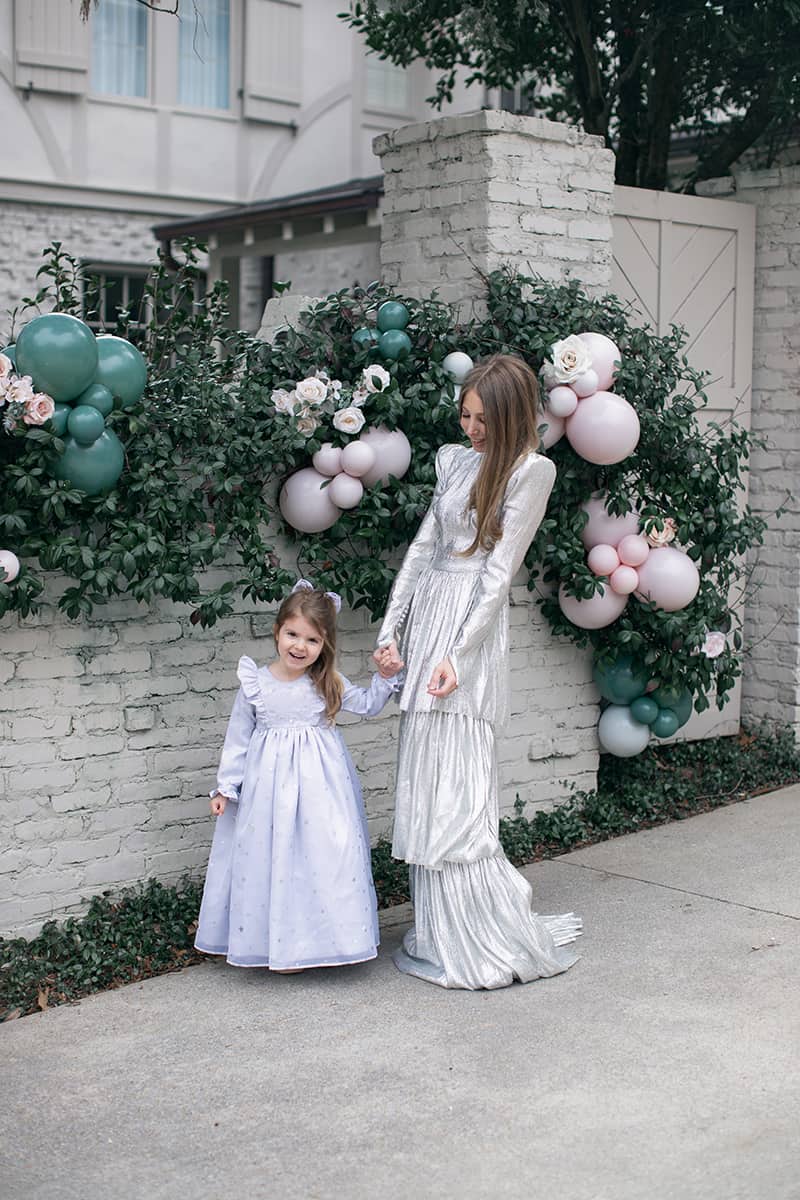In the picture, two girls are standing outside a well-maintained white building with a brick structure. They are on a concrete sidewalk adorned with a decorative arch made of pink and teal balloons interspersed with red roses and greenery. The arch is attached to a fence covered with lush plant life. One of the girls, appearing around three years old, is wearing a long white dress with ruffles around her shoulders and a purple bow in her dark brown hair, smiling at the camera. The older girl, about sixteen, stands beside her, holding her hand and looking down at the younger girl with a laugh. The older girl wears a layered, whitish-silver dress that covers her long brown hair and extends to the floor, suggestive of formal or event attire. The background reveals a white painted brick wall with windows and wooden shutters, along with a white wooden door. This picturesque scene hints at a celebration or special event, possibly a wedding.